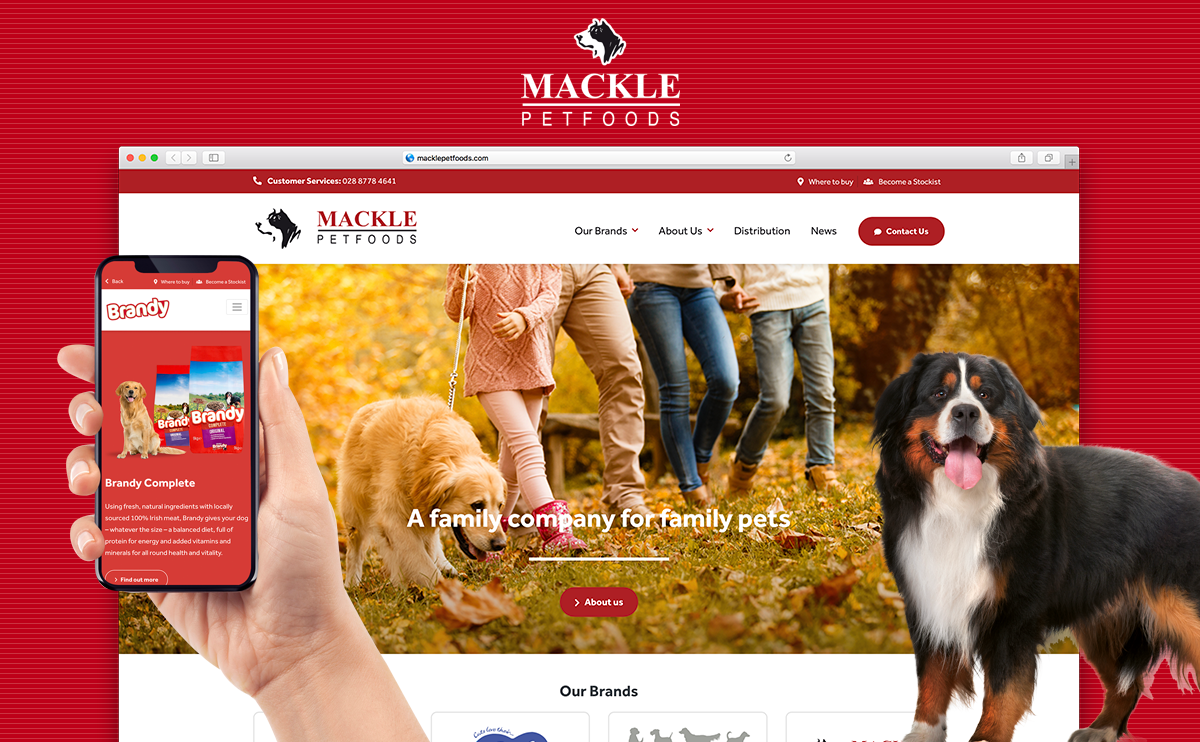This is a detailed description of a screenshot from the Mackle Pet Foods website. The screenshot prominently features the website’s interface, highlighted by a logo depicting a black and white Border Collie in side profile. Below the logo, "Mackle Pet Foods" is written in crisp white text against a textured background that transitions from burgundy to a lighter shade of burgundy horizontally.

At the top of the screenshot, typical internet browser controls are visible, along with the URL "macklepetfoods.com." The site’s navigation menu includes options such as "Customer Service" accompanied by the phone number 028 878 4646, "Our Brands," "About Us," "Distribution," "News," and "Contact Us." Additionally, there are features labeled "Where to Buy" with a GPS locator and "Become a Stockist."

The central part of the website's homepage showcases a background image of a family with their Golden Retriever, set in a picturesque autumn park. Adjacent to this image is another featuring a St. Bernard-like dog. A prominent banner displays the text "A Family Company for Family Pets." There is also an image of a hand holding a mobile phone, presumably to illustrate the website’s mobile-friendly design.